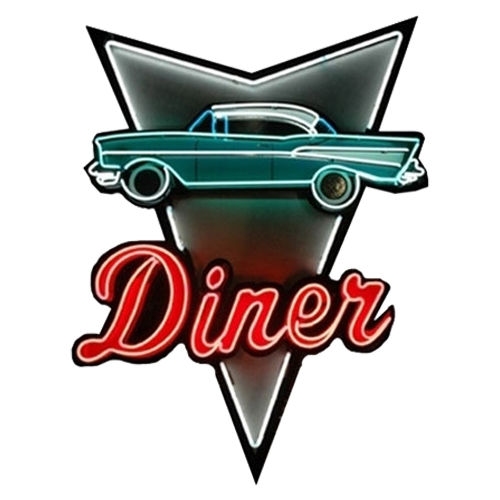The image resembles a visually striking decal or sticker, perfect for a diner advertisement. The design features an old-fashioned car, likely a 1950s model, with an eye-catching turquoise blue color and a white roof. The car is set against a white background and faces left. The entire image seems to have a neon glow, with a prominent white outline highlighting the details.

Beneath the car, in vibrant red cursive lettering, is the word "diner." Both the car and the word are set against a geometric shape resembling an upside-down triangle with an indentation at the top, giving it an arrow-like appearance. The borders of this shape are black, accentuated with white neon lights, adding to the overall vintage and inviting look of the sign.